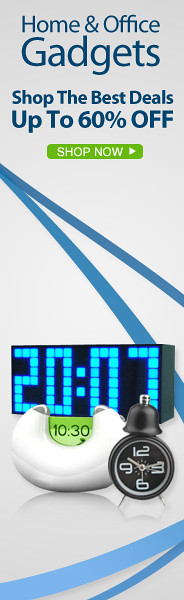This is a vertical rectangular-shaped ad on a gray background, promoting Home and Office Gadgets. At the top, it reads "Home and Office Gadgets" in blue font, followed by "Shop the best deals up to 60% off" in the same font. Below the text, there is a small green rectangle with "Shop Now" written in white, centered under the blue text. 

The ad features two intersecting blue lines at the top left, widening towards the center. Below this, there are three different clocks displayed. The first is a large digital rectangular clock displaying "2007" in blue digital light. The second is a round semi-circular clock with a small green face in the middle showing "10:30". The third is a small round analog clock with a bell on top, featuring white numbers for 12, 3, 6, and 9 on a black face, positioned towards the right. The arrangement of the clocks and the intersecting lines create a visually appealing layout.